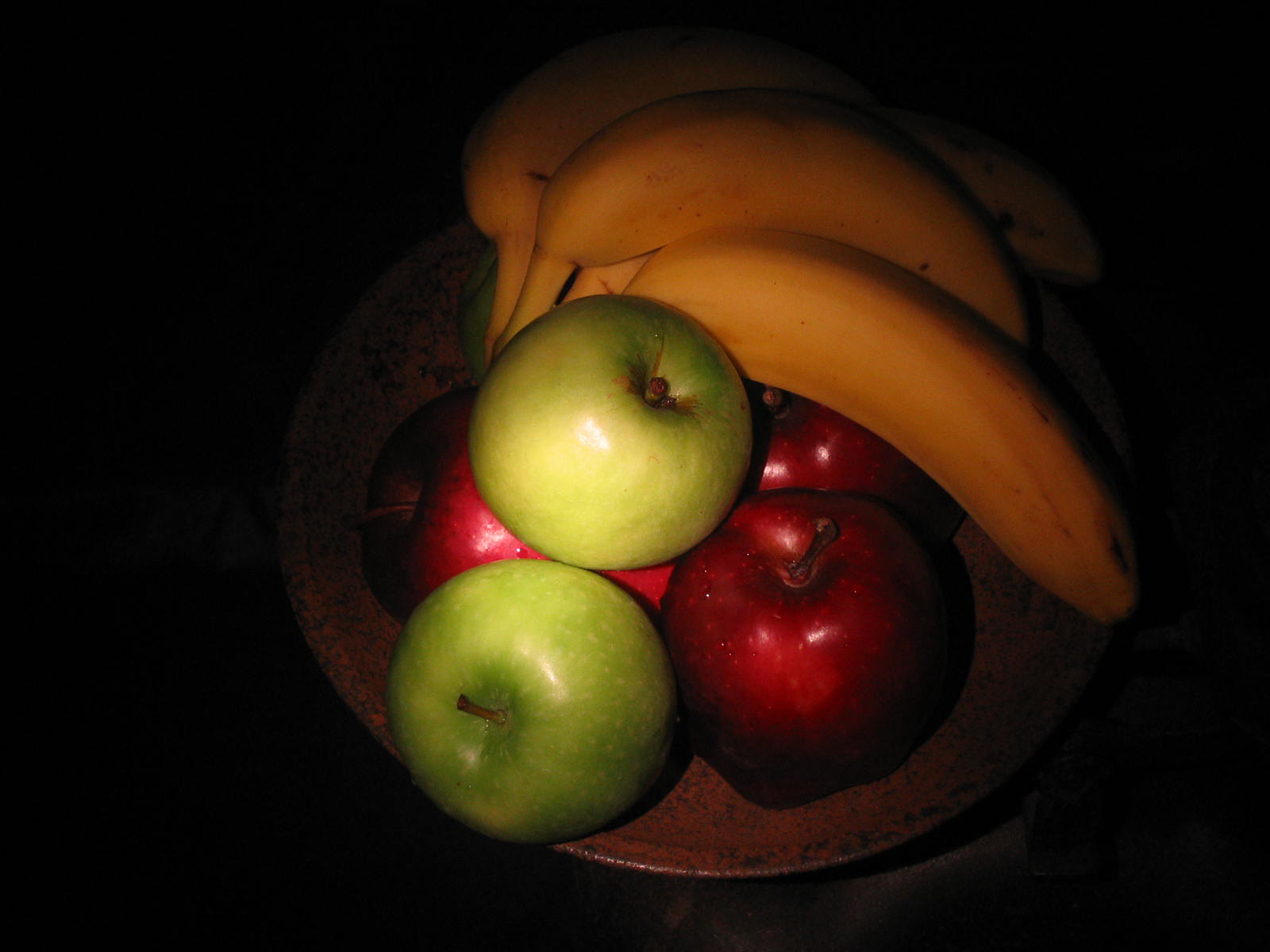In the dimly lit image, a wooden or possibly tarnished copper bowl brims with fresh fruit. The focal point is a trio of ripe bananas, all connected at the top stems, situated prominently at the bowl's rim. Nestled beneath these bananas are three vibrant red apples, their subtle sheen highlighting their ripeness. Lying atop these red apples are two green apples, equally mature and succulent. The low light conditions suggest that the camera's flash is the primary source of illumination, spotlighting the fruit against a shadowy background. The bananas, slightly cloaked in shadow, reveal their ripeness. Visible apple stems add to the authenticity and freshness of the display, making this bowl of fruit appear both inviting and naturally appealing.